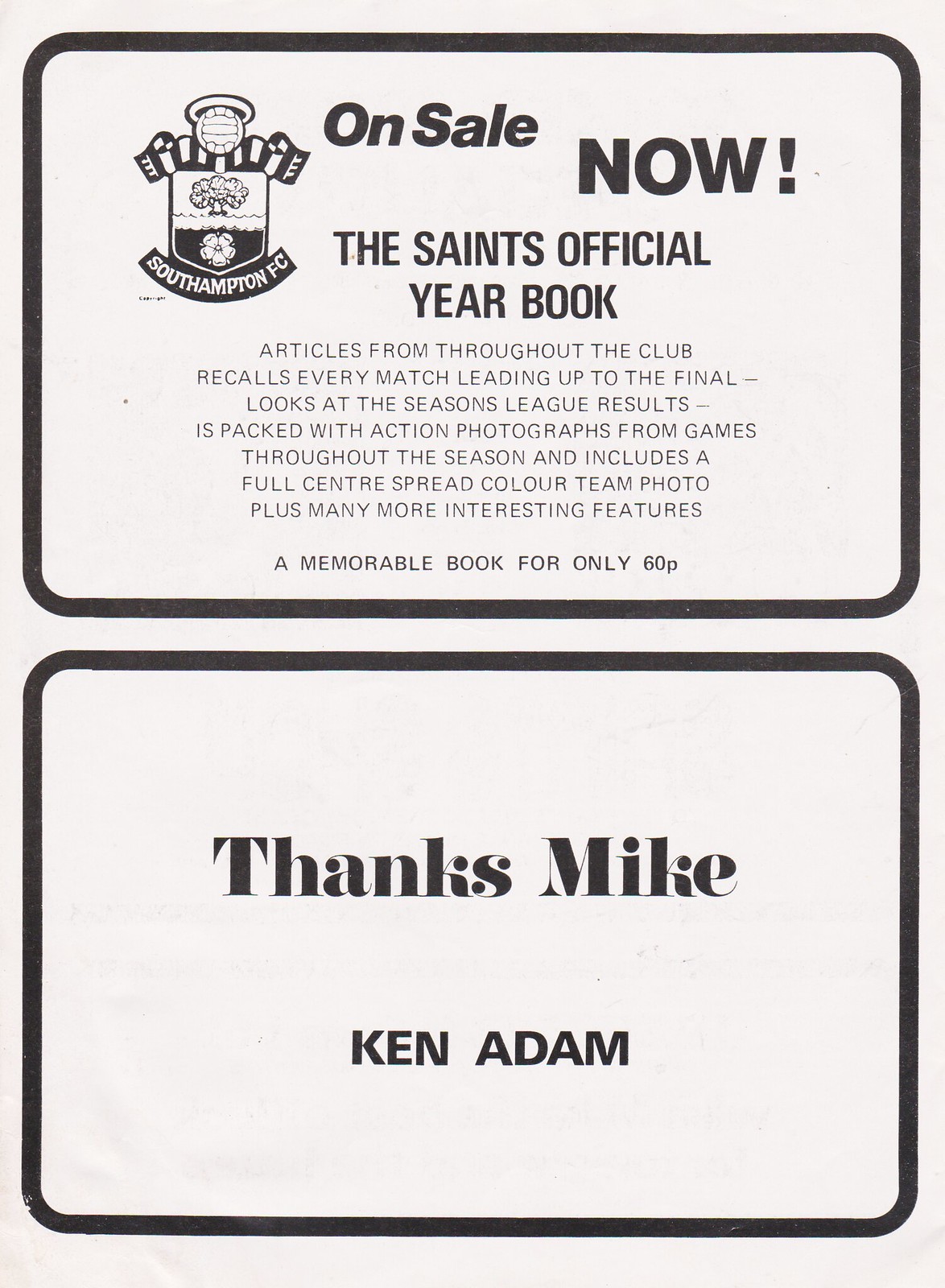The image features a piece of paper with a white background, divided into two rounded black rectangular frames. The top frame showcases the logo of Southampton Football Club on the left side. To the right of the logo, bold black text reads "On sale now!" with "on sale" in mixed capitalization and "now!" fully capitalized and punctuated with an exclamation mark. Below this, it says, "The Saints' Official Yearbook," followed by a detailed description boasting, "Articles from throughout the club, recalls every match leading up to the final, looks at the season's league results, is packed with action photographs from games throughout the season, and includes a full center spread color team photo, plus many more interesting features. A memorable book for only 60p."

The bottom frame, simpler in design, contains large bold black text in the center reading "Thanks Mike," and directly below, in a slightly different font, the name "Ken Adam."